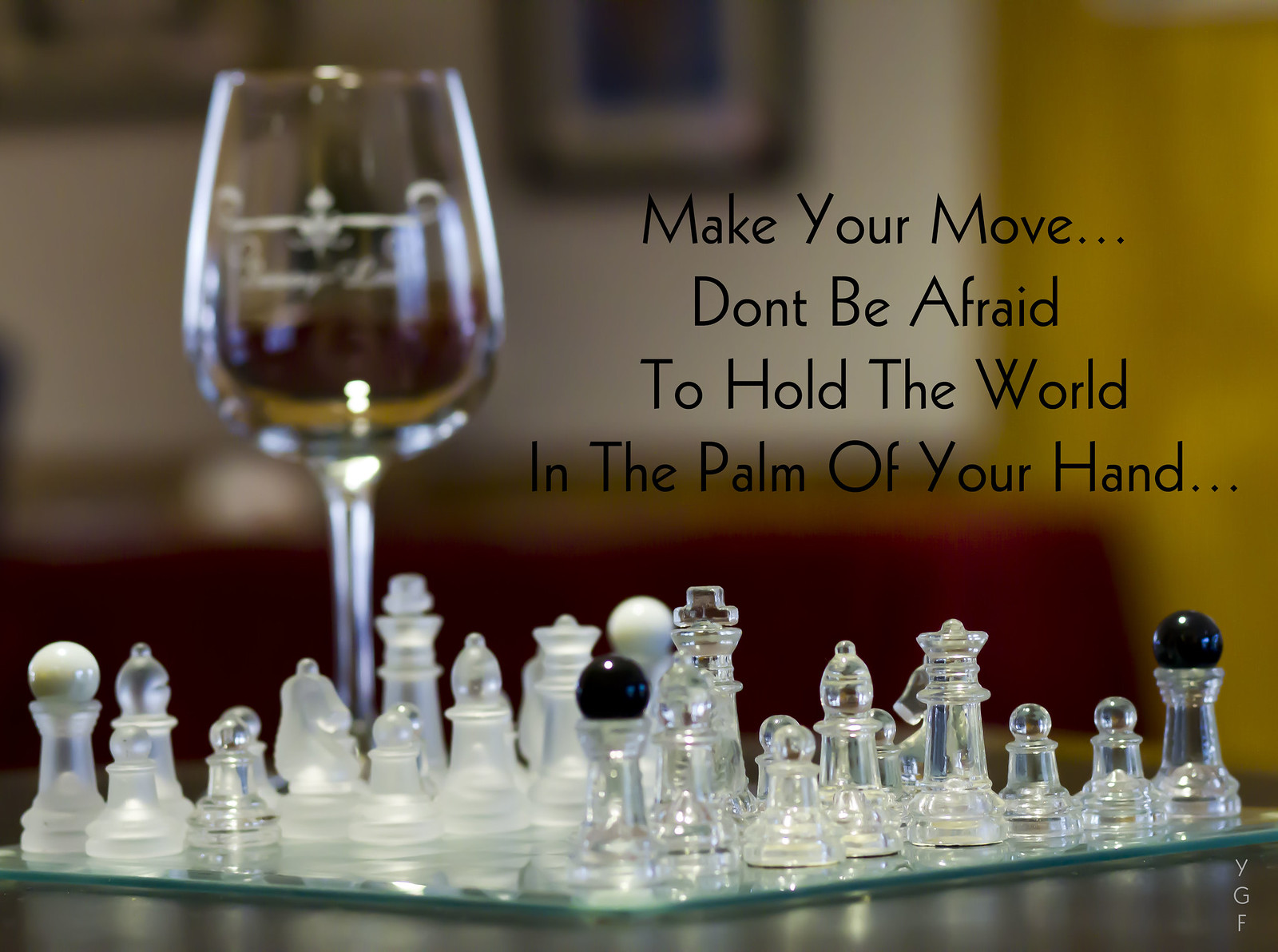This inspirational meme features a color photo of a small glass or crystal chess set, with the chess board made of either a mirror or a piece of beveled glass. The clear, transparent chess pieces are positioned on the right side, while the opposing set is crafted from translucent, frosted glass. Behind the chess set, slightly out of focus, is a wine glass filled with a brown liquid, possibly wine. The background is blurry, revealing a hint of a red sofa and a picture on the wall in the upper right corner. Bold black text overlays the upper part of the image, reading, "Make your move... don't be afraid to hold the world in the palm of your hand..." In the lower right corner, the initials "YGF" are also visible. The entire scene emphasizes the reflective quality of the glass chess board and pieces, adding depth and a sense of elegance to the composition.